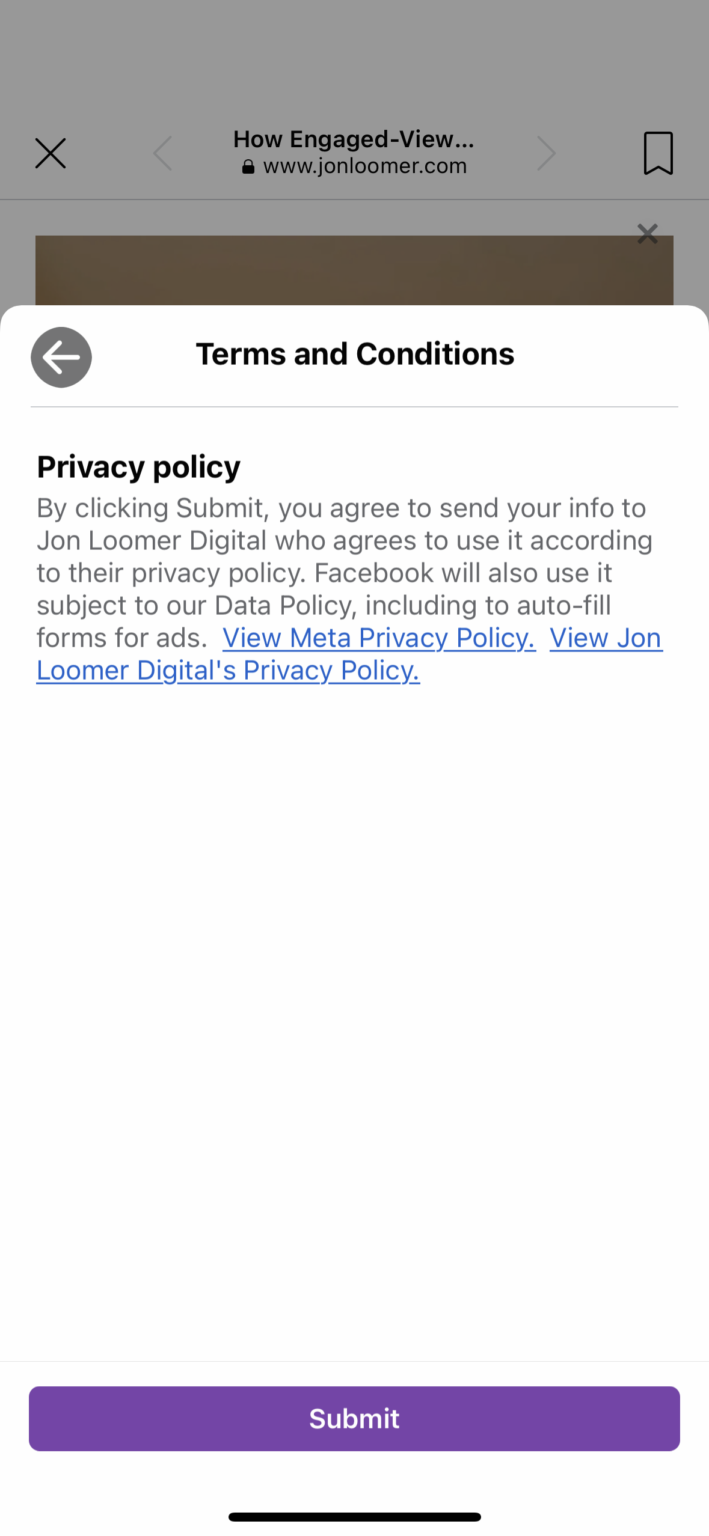The image displays a cell phone screenshot featuring a grayed-out background with a central overlay. At the top of the overlay, there is an "X" icon on the left corner, and next to it in the middle, it says "howengaged-view..." followed by a lock icon accompanied by "www.jonloomer.com" underneath.

The right side of the screenshot features a bookmark symbol at the top, with another "X" icon and a black box partially visible below it. The main focus of the screenshot is a white panel in the center displaying the terms and conditions, which cover the gray background previously described.

Within this panel, there is a back arrow key at the top left, followed by the title "Terms and Conditions." Below this, it mentions the "Privacy Policy" and includes a paragraph explaining the privacy policy. Toward the end of the text are two clickable links: "View Meta Privacy Policy" and "View John Loomer Digital Privacy Policy."

At the bottom of the screen, there is a purple background button with "Submit" written in white text.